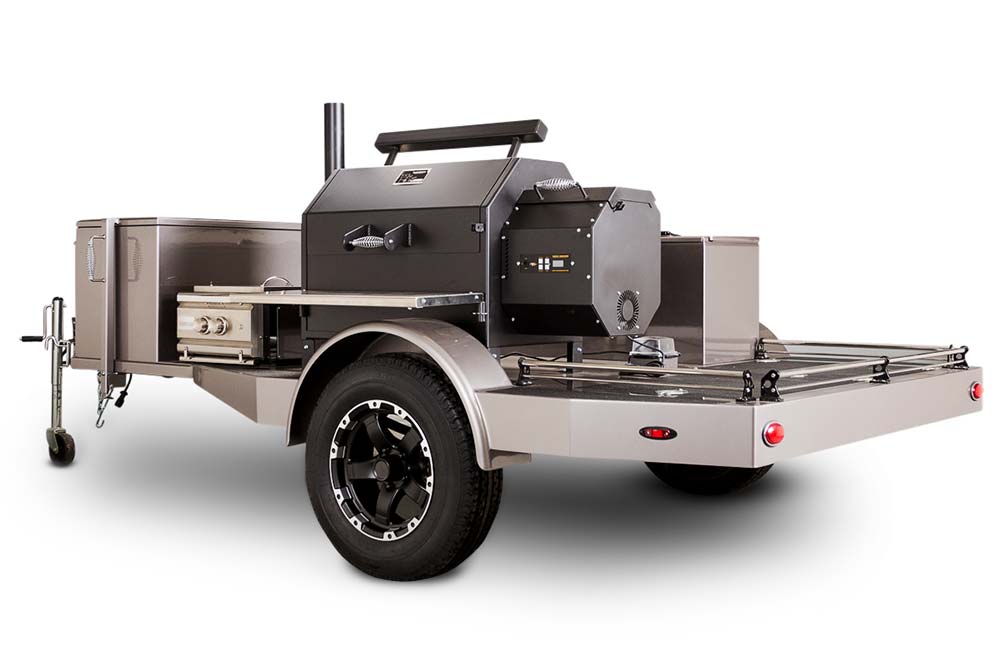The image depicts a shiny, silver, all-metal flatbed trailer with an organized barbecue setup on its surface. The trailer is equipped with massive, functional black tires featuring five-spoke hubcaps. Attached to the front of the trailer is a silver hook used for connecting it to a vehicle. At the front of the flatbed, there are two vertical rectangular metal cases with handles, likely used for storage. Immediately behind them lies a flat rectangular case. Dominating the center is a large black barbecue pit with a distinctive vertical rectangular shape and an arched top, accompanied by a black smokestack on the left. Adjacent to the barbecue is a secondary, more rounded compartment designed for smoking. Additionally, there is a cooktop with two burners and corresponding knobs, enhancing the trailer’s functionality as a mobile kitchen. The setup is further detailed with red lights at the rear, ensuring visibility.